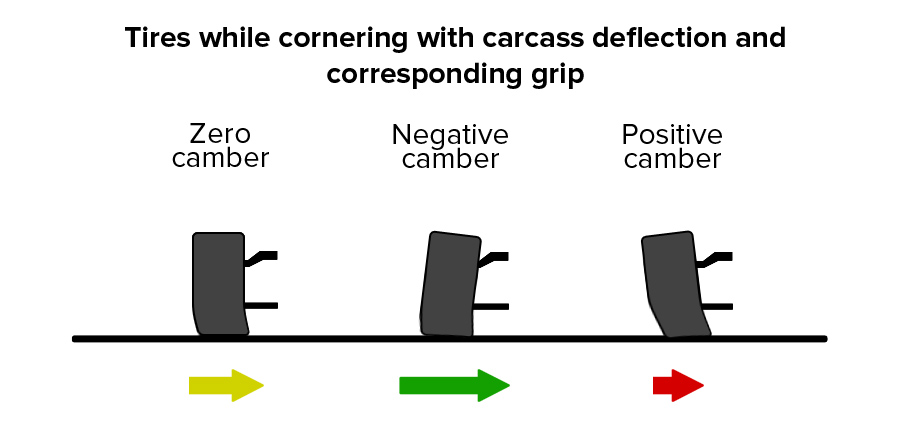This educational infographic, titled "Tires While Cornering with Carcass Deflection and Corresponding Grip," visually explains the different ways tire alignment affects grip during cornering. The infographic is divided into three sections, each illustrating a distinct tire alignment condition: Zero Camber, Negative Camber, and Positive Camber. 

- The "Zero Camber" section features an image of a tire with no tilt, labeled with a yellow arrow pointing to the right, indicating straight carcass deflection.
- The "Negative Camber" section shows a tire tilted inward at the top, supported by a green arrow pointed to the right, conveying increased grip through enhanced contact with the road during cornering.
- The "Positive Camber" section depicts a tire tilted outward at the top, highlighted by a red arrow pointing to the right, illustrating decreased grip due to reduced contact area with the road during cornering.

Each section is clearly labeled and color-coded to emphasize the differences in tire behavior and grip efficiency under varying camber conditions.